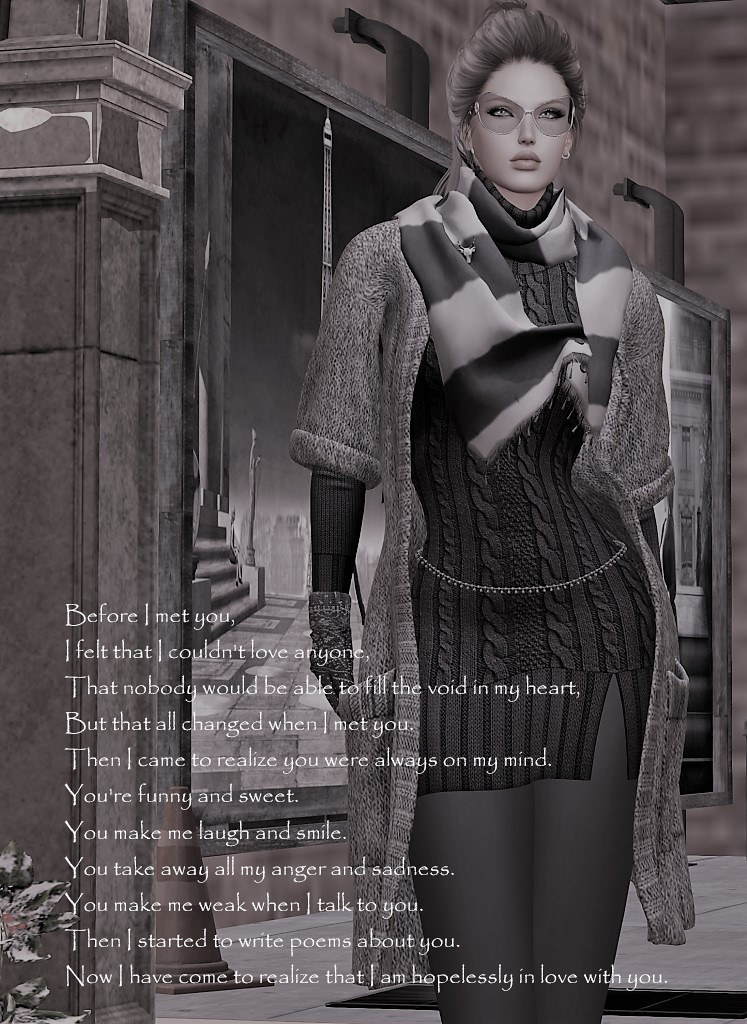In this black-and-white image, reminiscent of a video screenshot or an advertisement, a woman is standing upright on the right side, elegantly poised in front of a concrete building adorned with a partial cityscape mural featuring a tall spire and other buildings. She exudes confidence with her short, spiky, and professionally styled hair, reminiscent of a supermodel.

Her outfit is meticulous and fashionable: she wears a short sweater dress that reaches her upper thighs, paired with a long, light gray coat that extends below her knees. Around her waist is a delicate chain, adding a touch of elegance to her ensemble. The outfit is complemented by a striped scarf wrapped snugly around her neck, elbow-length sweater jacket sleeves, gloves, and leggings.

Accentuating her look are her teardrop eyeglasses, or possibly sunglasses, which add to her chic appearance along with her earrings. She has striking dark features that stand out against the grayscale background.

On the left bottom corner of the image, there is a poignant inscription in white text against a gray background. It reads: "Before I met you, I felt that I couldn't love anyone, that nobody would be able to fill the void in my heart. But all that changed when I met you. Then I came to realize you were always on my mind. You're funny and sweet. You make me laugh and smile. You take away all my anger and sadness. You make me weak when I talk to you. Then I started to write poems about you. Now I have come to realize that I am hopelessly in love with you." 

This thoughtful message, combined with the woman's sophisticated attire and the urban backdrop, creates a compelling and evocative image.